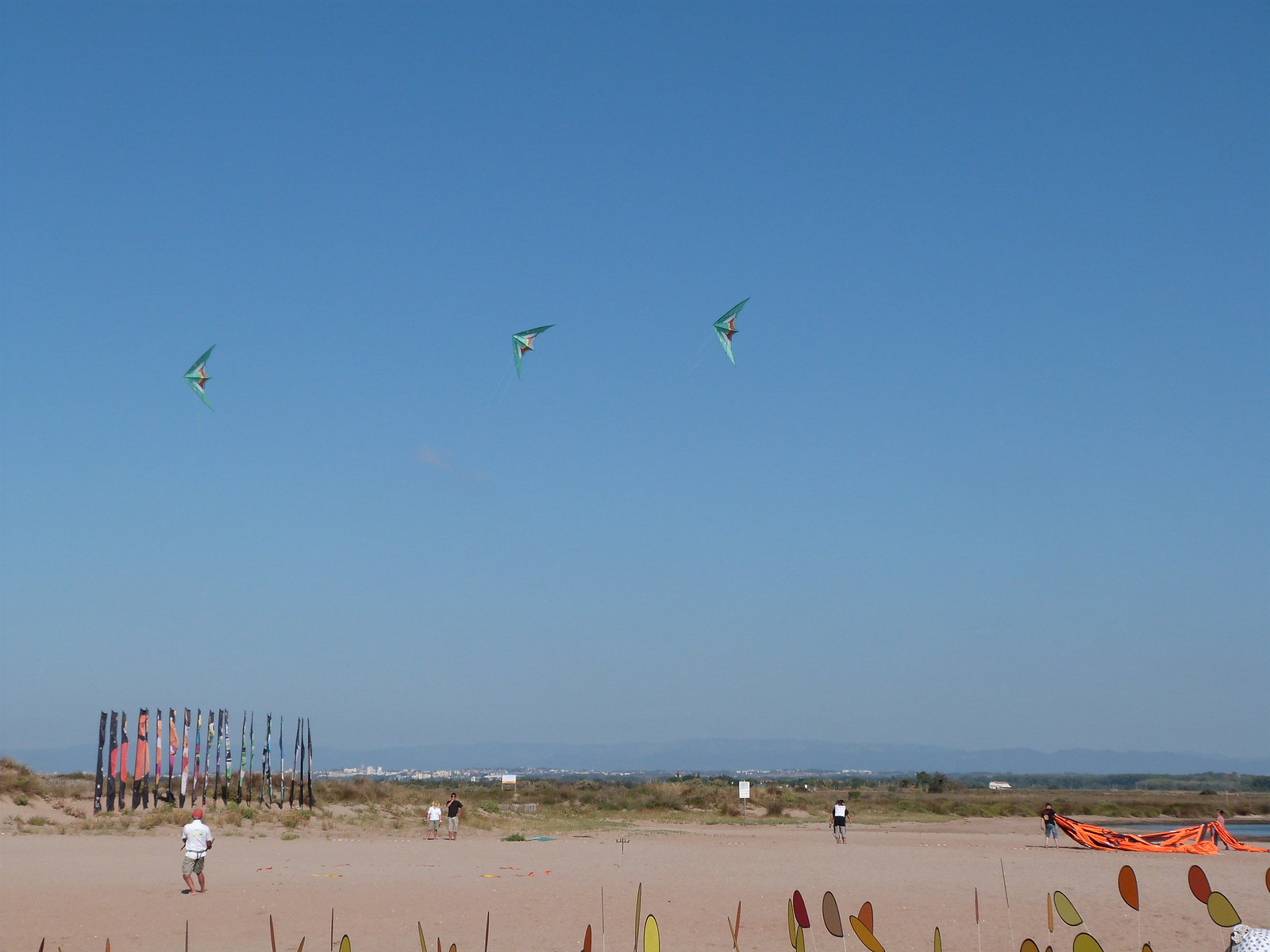In the foreground of this vibrant beach scene, a light brown sandy expanse sprawls across the bottom of the photograph, dotted with several people — most noticeable among them are two individuals in the bottom right, apparently struggling with a large piece of orange fabric or tarpaulin. On the left side, remnants of a wall consisting of long rectangular boards, possibly surfboards painted with artistic designs, protrude from the sand, arranged in a slightly spread-out manner. A few colorful blobs, red, yellow, and tan, possibly balloons or other objects, are scattered across the sand. Toward the rear of the beach, a shrubby, grassy area marks the transition from sand to vegetation.

Dominating the top portion of the image, a vast expanse of clear, blue sky stretches overhead. From the left side towards the middle, three triangular kites, each displaying a combination of blue, green, white, and possibly some yellow, soar in a perfectly aligned formation. These kites, looking somewhat like arrowheads, add a playful element to the serene sky, which features no visible clouds. In the distant background, the horizon faintly reveals the silhouette of mountains fading into the sky, and perhaps a glimpse of a shoreline with waves rolling gently in. White-shirted figures scattered across the sandy canvas appear like tiny specks, adding life to this picturesque seaside moment.